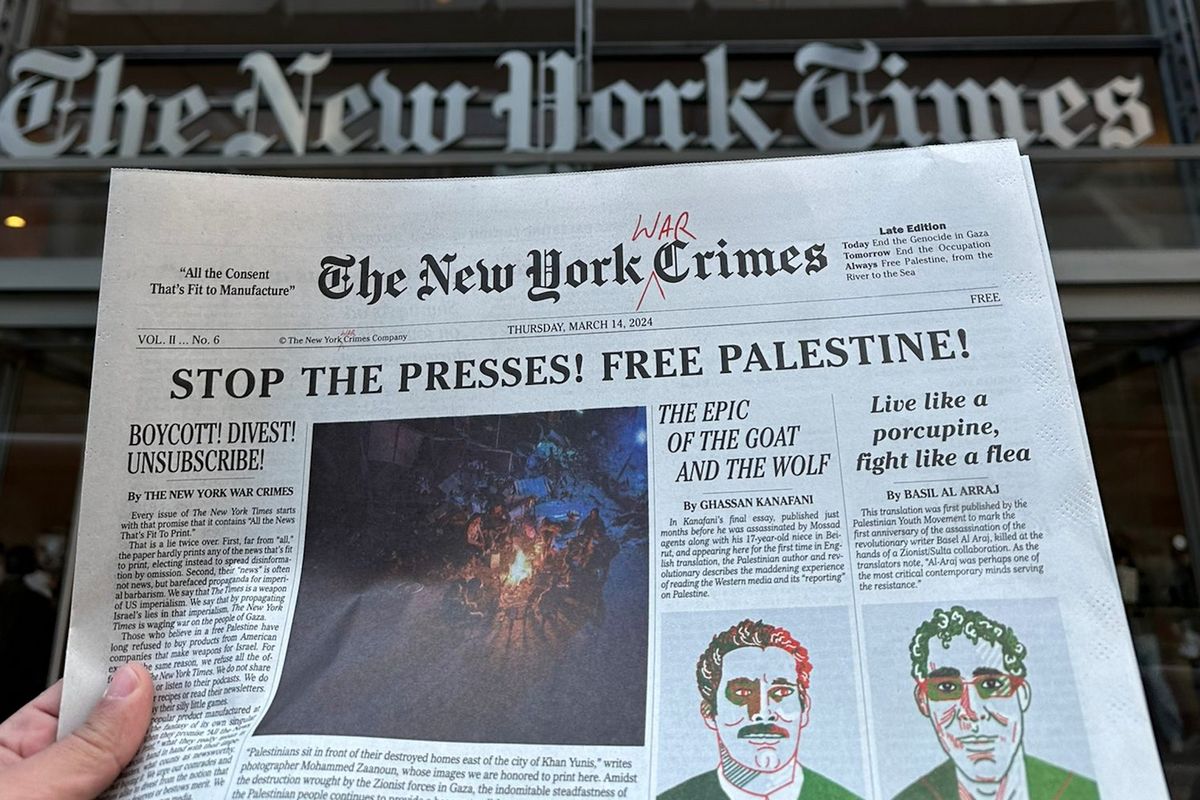In this image, we see a newspaper titled "The New York Times" prominently displayed. It is being held by a thumb and index finger on the left-hand side, with the thumb on top and the index finger below. Overlaid in red text, positioned to read "War Crimes," is the word "war" with an arrow pointing after "Times." The masthead specifies the date as Thursday, March 14th, 2024, with the word "free" appearing on the right-hand side.

Below the masthead is a striking call to action: "Stop the presses! Free Palestine!" with an emphatic tone conveyed through exclamation points. The page features an illustration of what appears to be a campfire against a blue background, with two sketched individuals colored in green and red beneath it. Further down are slogans such as "Live like a porcupine, fight like a flea," and "Boycott, divest, unsubscribe." Above the newspaper, there is a laminated "New York Times" logo superimposed on a building, enhancing the image's layered narrative. The entire scene suggests a strong protest message advocating for political causes, particularly related to events outside the U.S.